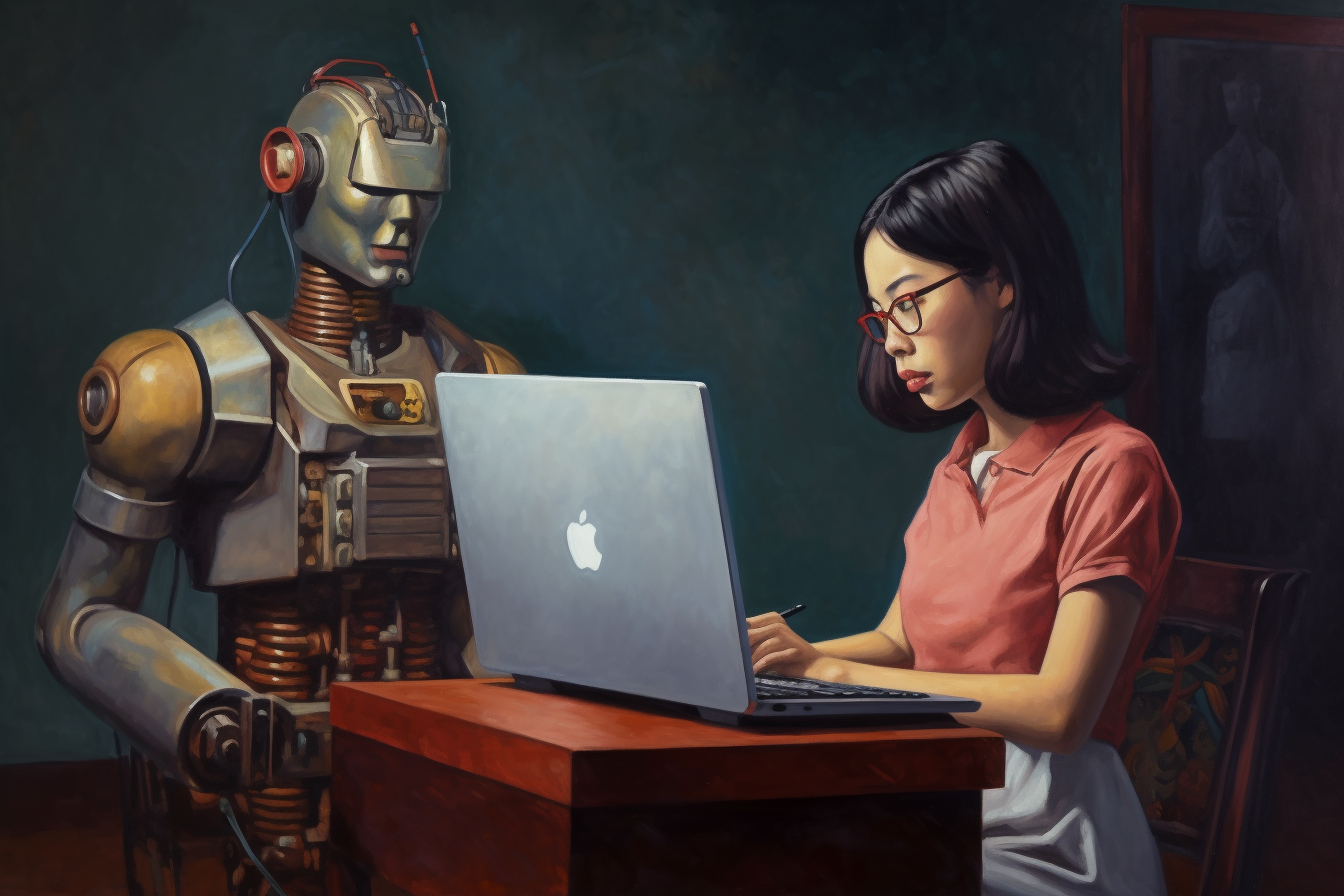In this detailed painting, we see an Asian woman with dark black hair, wearing red glasses and a light pink shirt. She is sitting at a dark mahogany brown desk, focused intently on typing on her silver Apple laptop. The woman, who looks cute and studious, also has a white skirt and gray bottoms, suggesting a well-coordinated outfit. 

To the right of her stands a futuristic and intricately designed robot, featuring a mix of silver, brown, and rusty golden colors. The robot, which appears slightly aged with elements like coils and an antenna, has visible componentry and machinery, showcasing a blend of both modern and vintage aesthetics. Some of its parts, including an ear-like shape, are red, adding to its complex appearance.

The background of the scene is dark green with hints of blue and light cascading down from the top, casting a soft glow on the subjects. Behind the woman, there's a portrait of an indistinguishable figure, contributing to the painting's mysterious ambiance. The entire setting combines elements of realism and a cartoon-like quality, making the image both captivating and intriguing.